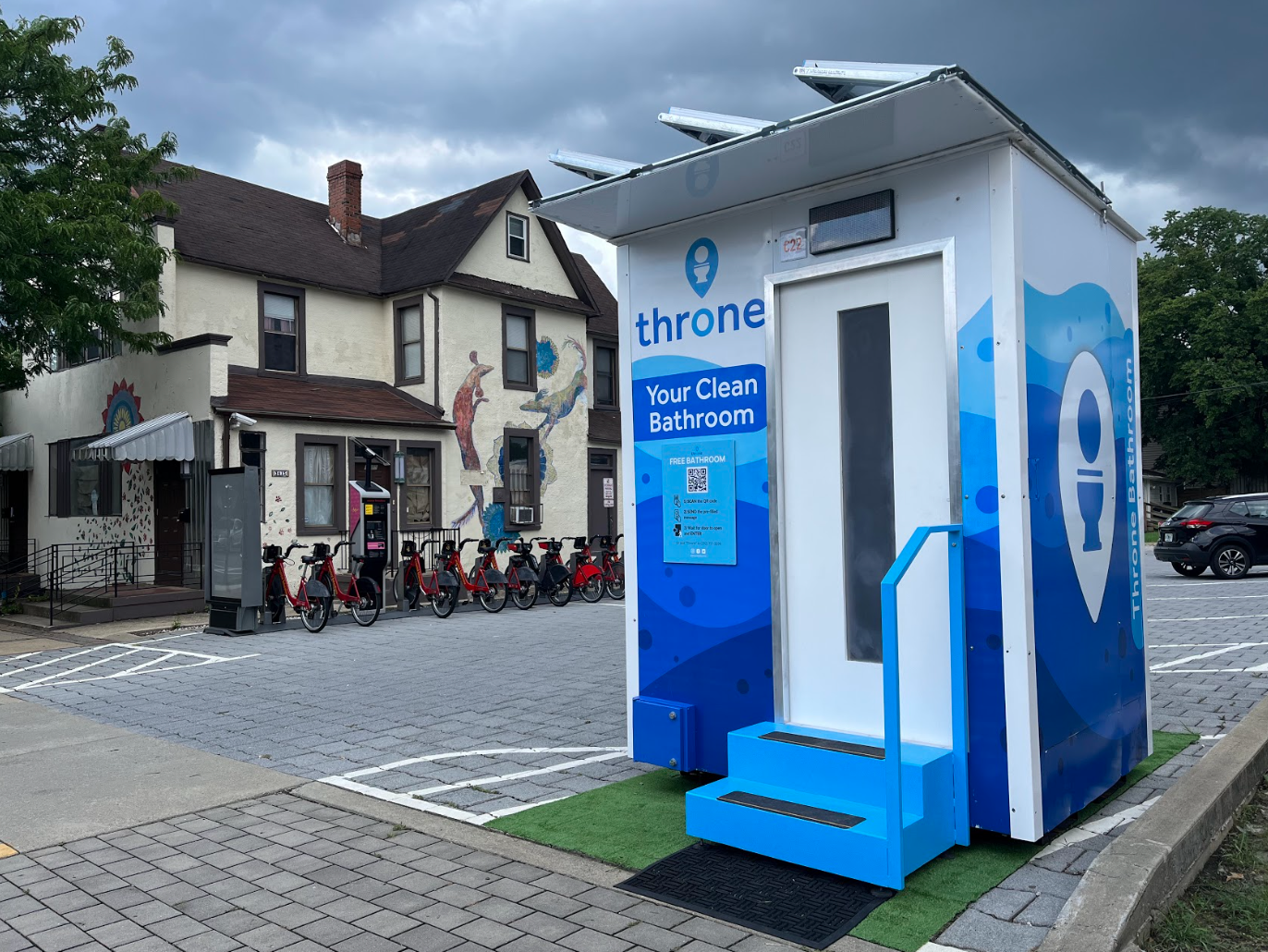In an outdoor scene, a blue and white portable toilet, marked with the brand "Throne," stands on a small patch of artificial grass in the foreground, right side. This modern, self-cleaning bathroom features a white door with an obscured window and blue steps, and it advertises itself with the slogan "Your clean bathroom" alongside a toilet logo. A QR code and some instructional posters are visible, indicating how to use the facility.

The background reveals a parking lot paved with gray cobblestone bricks, where multiple rental bikes or scooters, primarily red, are lined up beside a large building. This two-story establishment, possibly a restaurant or pub, has tan walls, a slanted shingled roof, and a chimney. It is adorned with mural paintings on one section and features two canopies at the front. Cars are parked nearby, including a black car, adding to the bustling yet organized atmosphere, even under the cloudy sky.